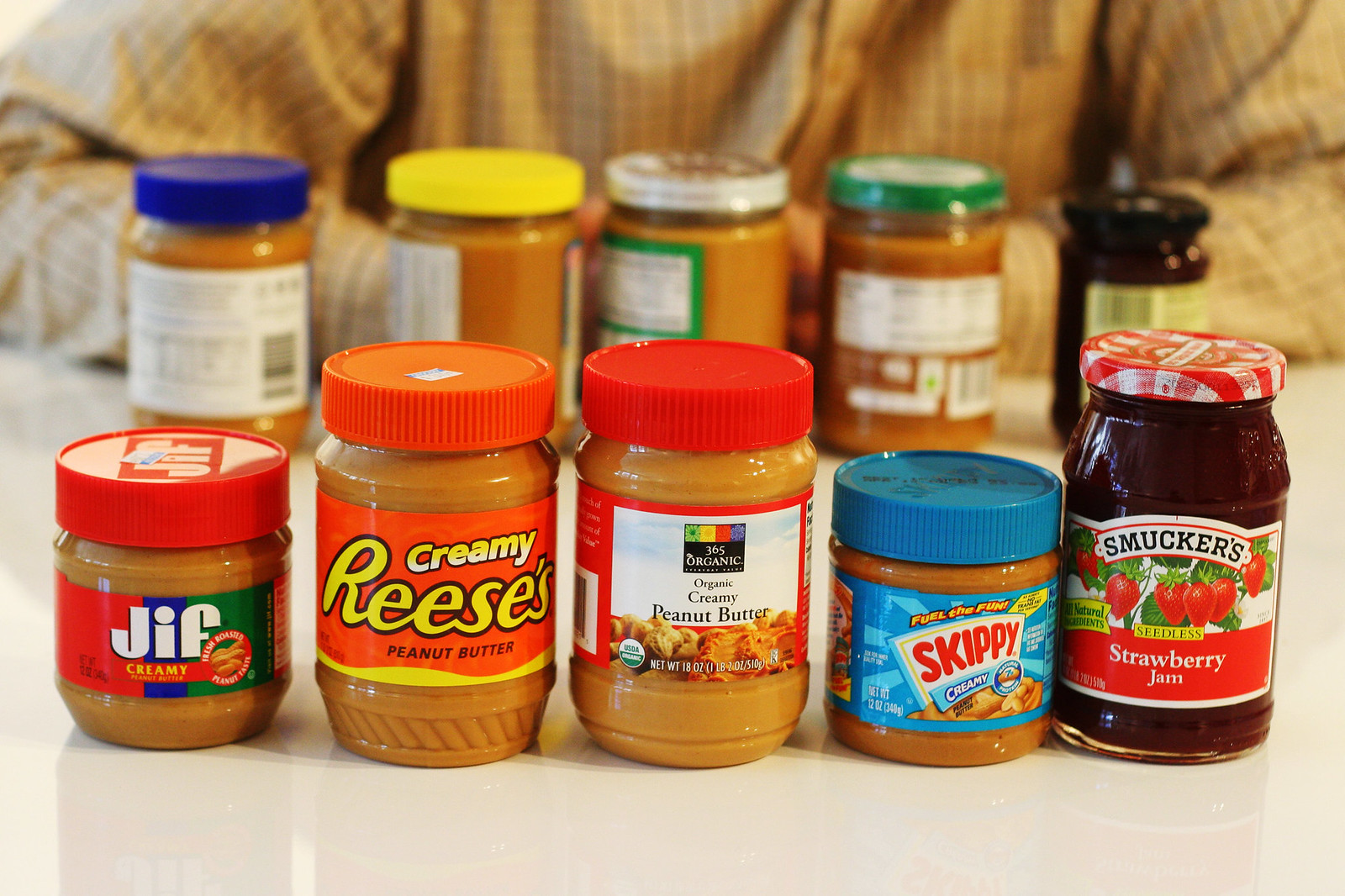This image showcases a variety of peanut butter and jelly jars arranged on a white table. In the foreground, five jars are positioned with their labels facing the camera: a small jar of Jif creamy peanut butter with a red lid, a large Reese's creamy peanut butter jar with an orange lid, an organic creamy peanut butter jar with a red lid, a small Skippy creamy peanut butter jar with a blue lid, and a Smucker's strawberry jam jar with a red and white checkered lid. Behind this front row, there is another row of jars, turned so their labels are not visible. This back row includes jars with lids of blue, yellow, silver, and green with white inside, along with an additional jar of dark purple jam or jelly with a black lid. The background features the torso of a person, wearing a brown and white checkered or striped shirt, who appears to be leaning on the table, creating an off-white surface for the display. Their forearms and hands are visible, positioned at a 90-degree angle.